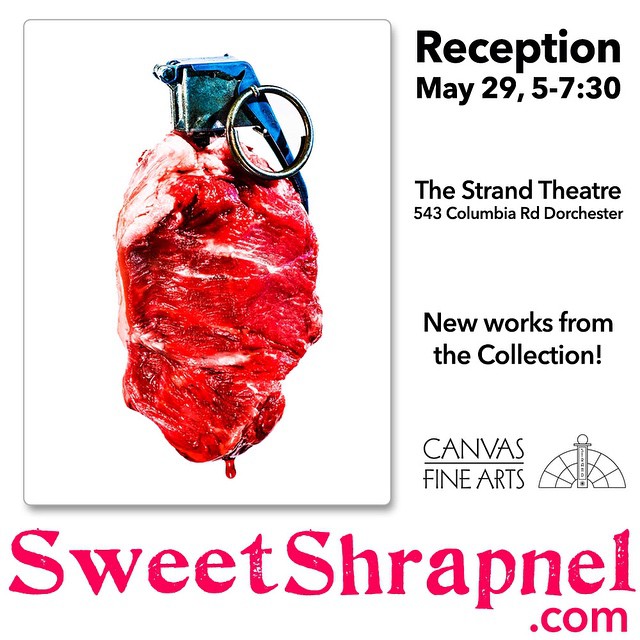The advertisement for the art fair is visually striking with a white background. Dominating the left side of the image is a vivid illustration of a piece of steak with the top handle of a red grenade thrust into it. The silver round pin of the grenade handle is still attached, and there's a single drop of red blood dripping from the bottom of the steak. This central image captures attention with its bold use of color and provocative design. 

To the right of this image, the event details are clearly displayed in bold black letters: "RECEPTION MAY 29, 5-7:30 PM". Below this, the venue is listed: "THE STRAND THEATRE, 543 COLUMBIA ROAD, DORCHESTER." Further down the text reads "NEW WORKS FROM THE COLLECTION!" Underneath these details is the name of the organizing body, "CANVAS FINE ARTS", accompanied by a distinctive logo that resembles a barometer with a rainbow-shaped window behind it.

At the bottom of the advertisement, spanning the width in bright pink letters, is the website: "SweetShrapnel.com". This comprehensive blend of imagery and text provides a compelling notice for the upcoming reception on May 29th, inviting viewers to see new artistic works at the Strand Theatre.